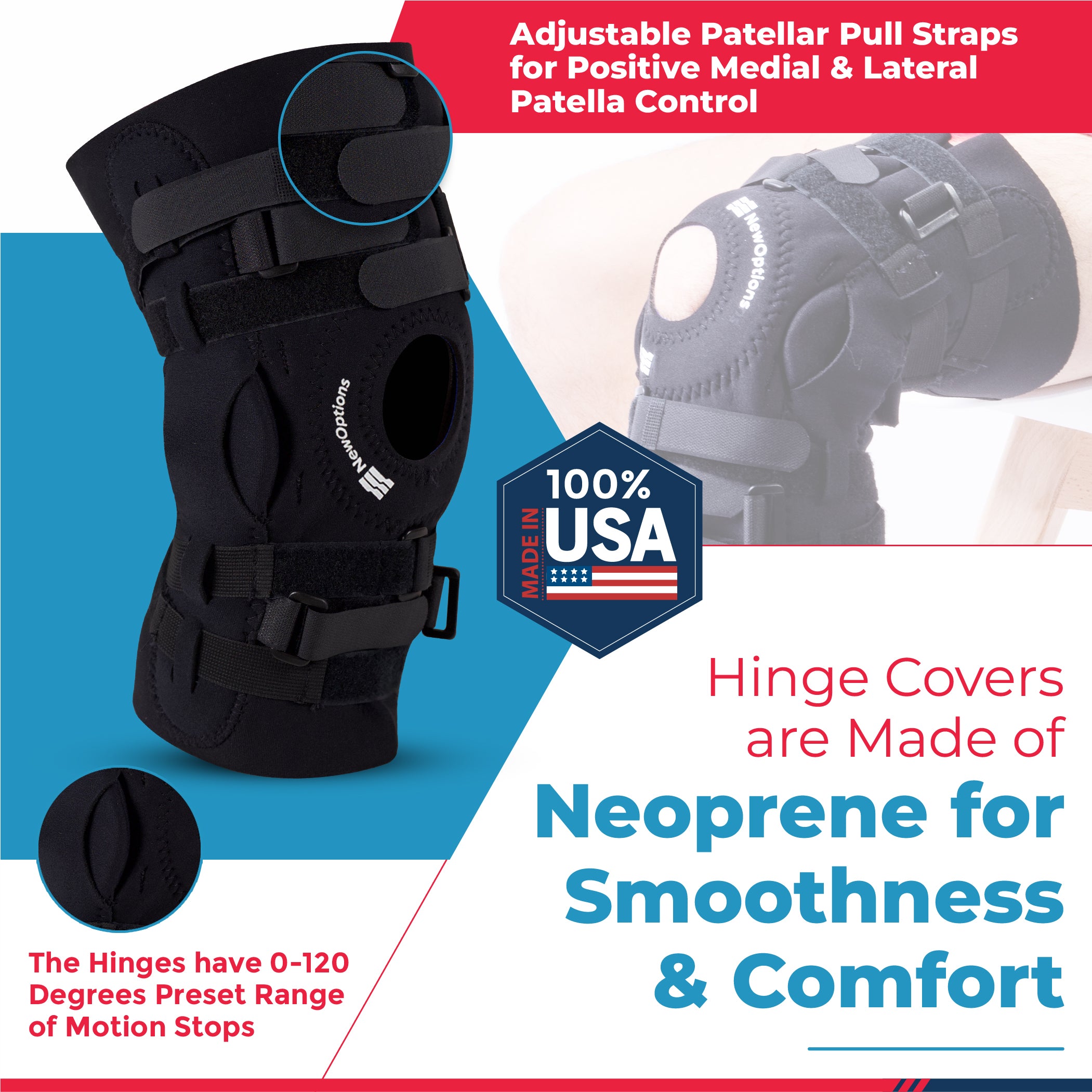The advertisement showcases a black knee brace, crafted from neoprene material, with a focus on comfort and functionality. Prominently displayed on the left side of the image, the knee brace features Velcro straps at the top for secure attachment and a central opening around the knee area labeled "New Options." Notably, the adjustable patellar pull straps are designed for positive medial and lateral patella control. The advertisement emphasizes the quality and origin of the product with the text "100% made in the USA," accompanied by an American flag. The hinges of the brace provide a preset range of motion stops from 0 to 120 degrees, ensuring customizable support. Additionally, the hinge covers are made from neoprene to guarantee smoothness and comfort. A red and blue border frames the bottom of the advertisement, adding to the overall aesthetic. In the background, a blue and white color scheme enhances the professional appearance of the ad.